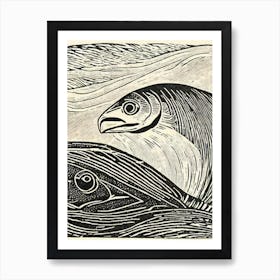The image is a black and white artwork, framed with a black outer frame and an inner white border. The art piece itself is rectangular and presented on a white wall. Within the artwork, a detailed drawing primarily depicts the head of a fish, featuring black eyes and a distinct black top with a matching black body. The fish appears to be emerging or interacting with an abstract element that might represent a wave or another shape. The ambiguity of the scene has led to interpretations of the fish resembling other creatures, such as an elephant with a fish head, suggesting a surreal or imaginative composition. The overall appearance of the artwork, drawn with a pencil-like texture, contributes to its abstract and unclear nature, leaving its exact depiction open to viewer interpretation.